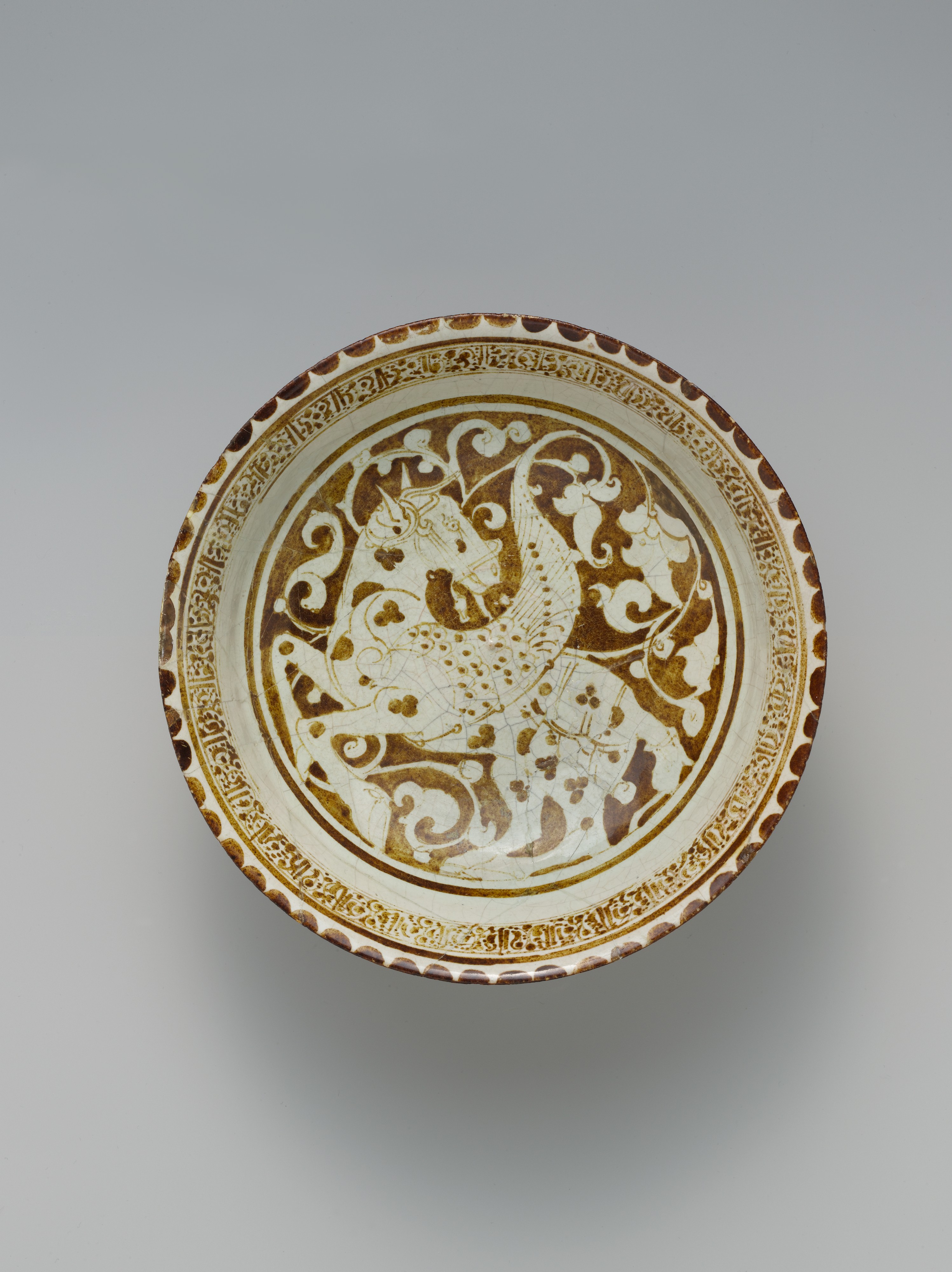The image captures an intricately designed porcelain bowl in an aerial shot. The background of the photo is a light gray. The bowl, predominantly white with brown and gold accents, showcases a central image of a mythical winged horse, adorned with horns and surrounded by flowering vines. This central artwork sits on a brownish-gold background and is bordered by a gold circle. Ascending towards the bowl's rim, there are concentric circles: a white band, followed by a patterned brown band, and finally, the rim adorned with brown semicircles. The detailed interplay of floral designs and concentric patterns adds to the bowl’s elaborate craftsmanship.